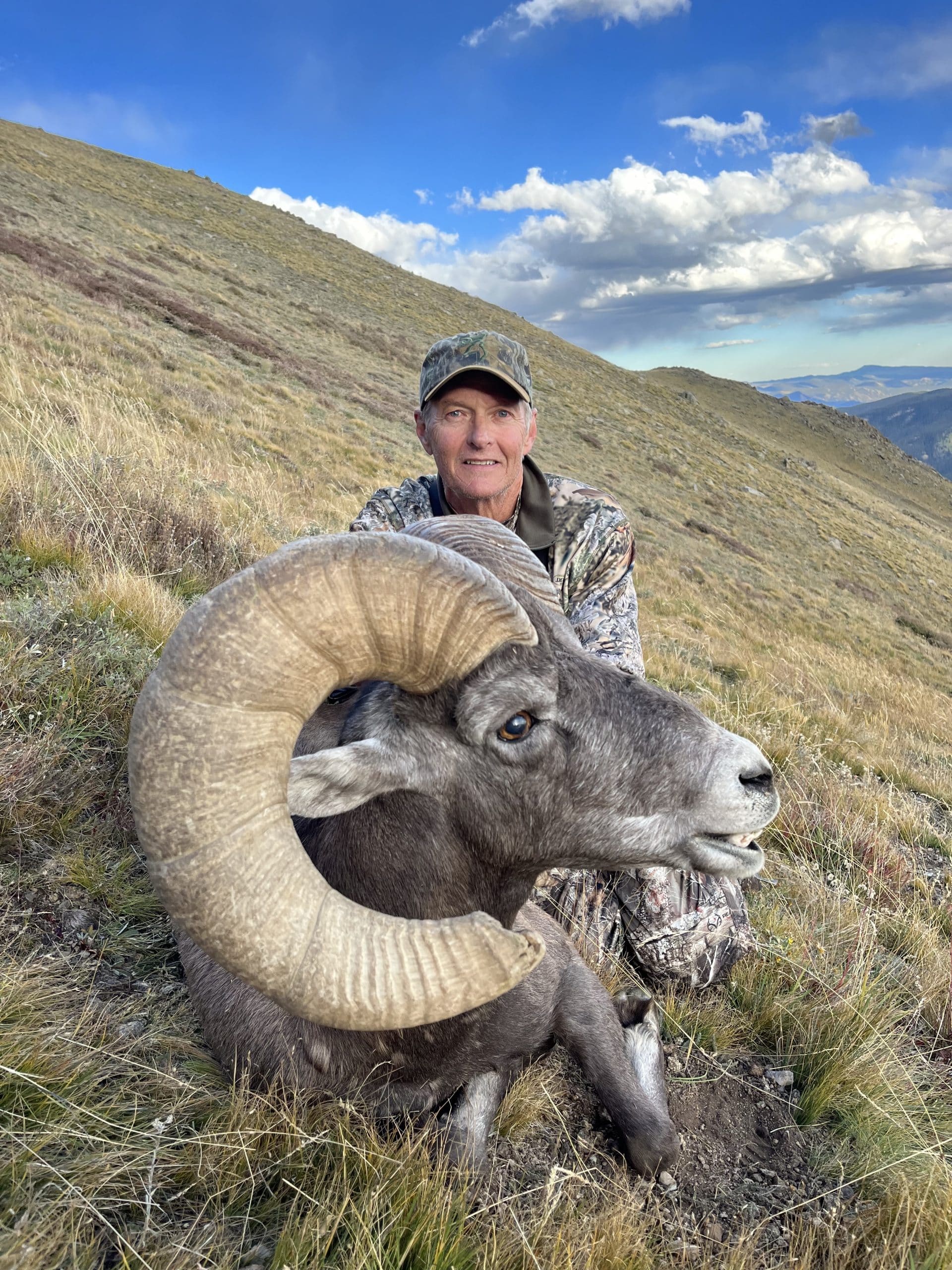An older man, likely in his 60s with white hair peeking from under his camouflage hat, is sitting on a grassy hillside under a mostly blue sky with a few clouds. He is dressed head-to-toe in greenish-gray camouflage, smiling as he poses beside a large ram that he appears to have hunted. The hillside, which slopes downward to the right, is mostly covered in brown straw-like grass with minimal green vegetation, suggesting a mountainous location. The ram, with its massive curling horns extending near its chin, lies in a defeated position with its legs folded beneath it. It has a grayish-brown coat with hints of white. The setting is serene with a clear day, the sky predominantly blue on the left side but thicker clouds gathering toward the right.